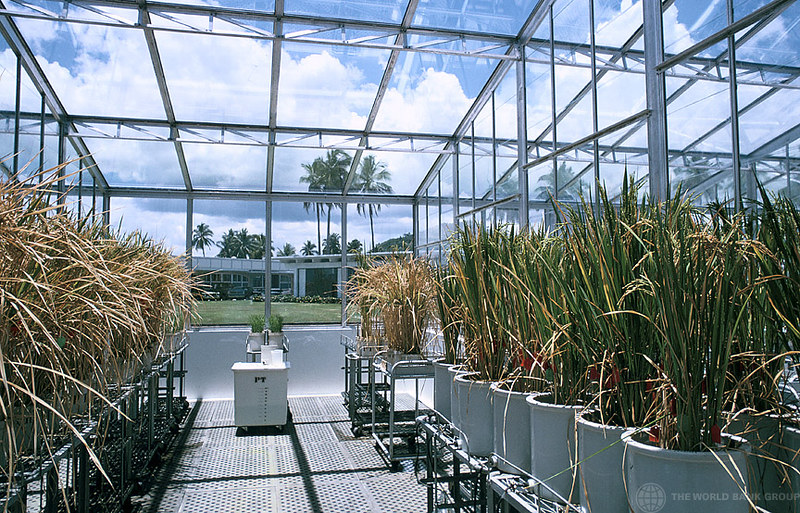The photograph depicts a sunlit greenhouse with windowed walls made of glass panels supported by metal frames. Inside, there are rows of plants, some of which appear healthier than others. The left-hand side features plants growing directly in the ground or dirt, possibly already harvested. The right side consists of plants in blue ceramic pots with red tags, displaying lush green foliage. Smaller green plants are positioned centrally, and a white machine is visible mid-room. The floor has a grating system likely used for drainage. Outside the greenhouse, palm trees and fluffy clouds suggest a tropical climate. In the distance, a house can be observed. The bottom right corner of the image displays the World Bank Group logo featuring a globe and a World Wide Web icon.